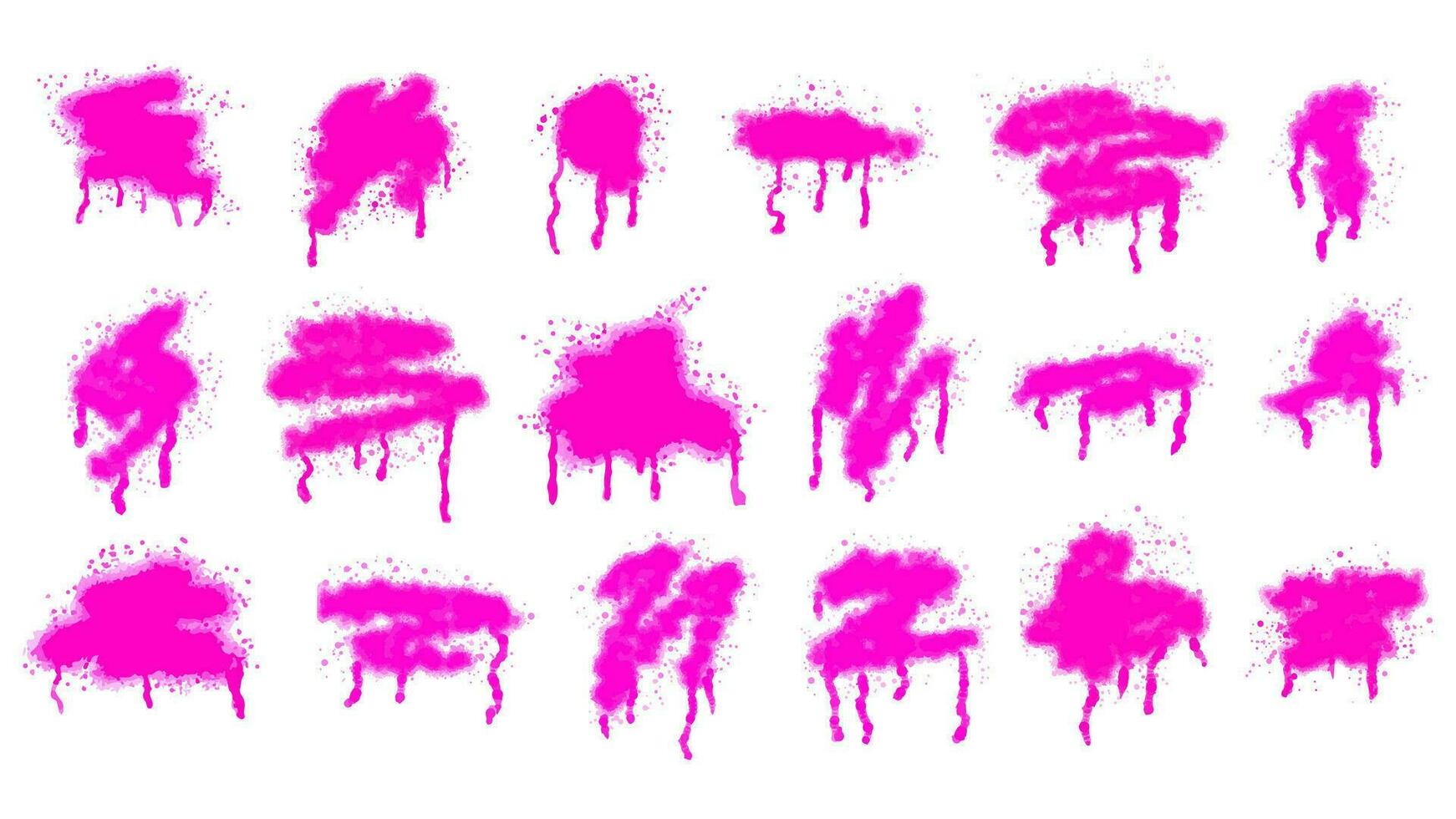The image is a digital abstract painting featuring 18 distinct splotches of hot pink spray paint, meticulously arranged in a grid against a pure white background. The grid comprises six columns and three rows, with each cell containing a unique pattern of paint. Each splotch exhibits a variety of shapes—some resemble letters like 'Z' and 'N', others appear like symbols or random shapes often likened to graffiti. All the paint splotches present small dotted areas around the main blotch, with rivulets of paint running down, emphasizing the dripping spray paint effect. Some shapes are horizontal sprays, some vertical, and some form circular patterns, adding a sense of dynamic randomness to the composed layout.